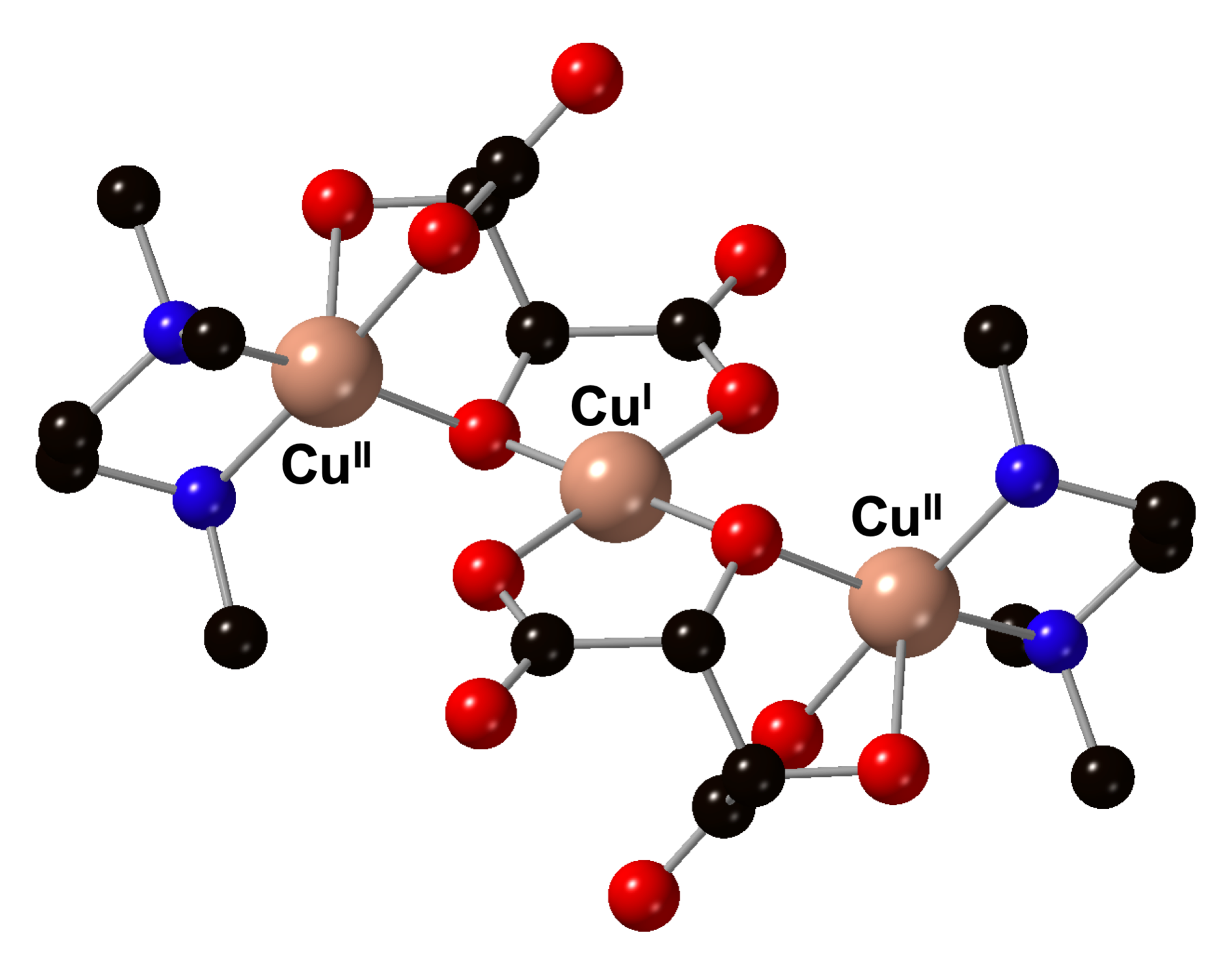The image is an animated, three-dimensional representation of a molecular structure set against a white background. The central feature of the molecule consists of three large, shiny, copper-brown spheres. Each of these spheres is labeled with the notation "Cu," followed by small Roman numerals I or II (I, II, or II). These copper-brown spheres form the core of the structure and are each connected to several smaller, multicolored balls via thin, silver-gray sticks that resemble sewing pins without heads.

These smaller spheres come in four distinct colors: red, black, blue, and a dark tan or light brown. The red and black spheres dominate the structure, with several of them connected directly to the copper-brown spheres. Blue spheres are less frequent, with only four visible in the entire structure—two at the top and two at the bottom. Each smaller sphere also connects to other multicolored spheres through the same thin silver-gray connectors, creating a complex, web-like network that reflects a detailed, scientific visualization of the molecule in space. All parts of the molecule are slightly glossy, enhancing the visual depiction of the structure.